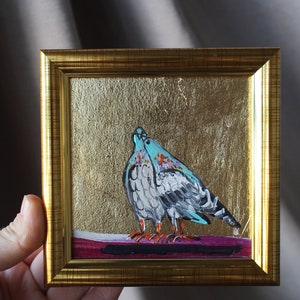This is a square photograph capturing a very small, intricately detailed painting. The painting, securely held by a fair-skinned hand visible in the bottom left of the image, is encased in an elegant yet simple gold frame, roughly four inches wide. The artwork itself features a striking gold foil background with a burgundy lower section that takes up about 10% of the composition. Atop the burgundy platform, which has been described as pink by some, stand two teal-colored birds that are likely lovebirds. The bird on the left stands tall, while the bird on the right leans in affectionately, appearing to nuzzle against its mate. Details include their teal bodies with white and black wings, and vivid orange claws. The rich, metallic gold background imparts an expensive and shiny appearance, enhancing the overall visual appeal of this exquisite miniature painting.